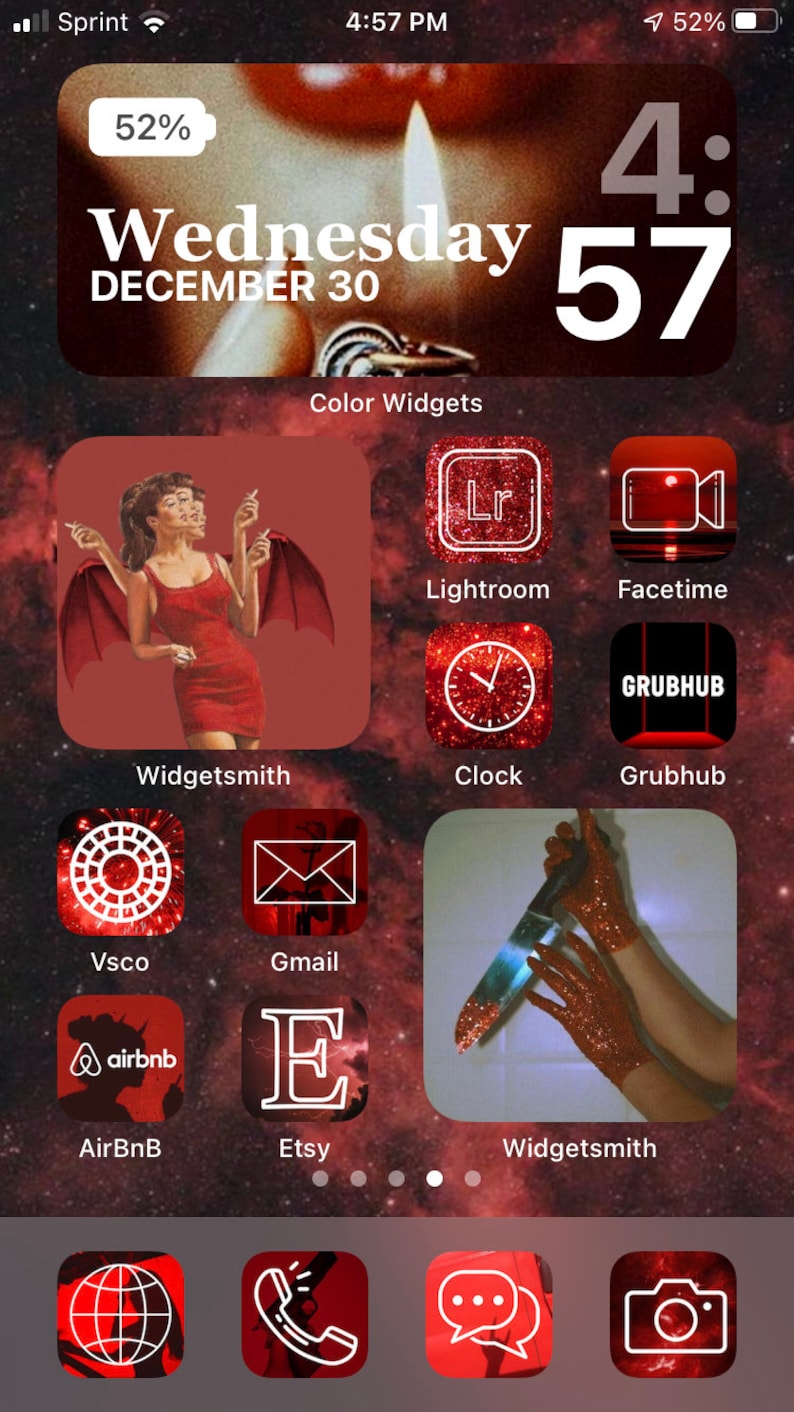This screenshot, taken on an Apple iPhone with Sprint service, captures the device in use at 4:57 PM with 52% battery life remaining and connected to Wi-Fi. The home screen features a visually striking, gothic-themed design dominated by red hues and fantasy elements inspired by Dracula.

The first widget prominently displays a close-up of a woman's lips with a flame flickering in front of them, set against the backdrop of the current date and time, Wednesday, December 30th, 4:57 PM. Below this is a second widget portraying a woman adorned with Dracula wings, enhancing the vampiric aesthetic. The third widget showcases a pair of hands wearing red glittery gloves, gripping a large chopping knife, adding a macabre touch to the screen.

All the visible app icons are customized to fit the red theme, including commonly used apps such as Safari, Phone, Messaging, Camera, and Etsy, which features a red icon with white contrast, seamlessly blending into the overall gothic ambiance.